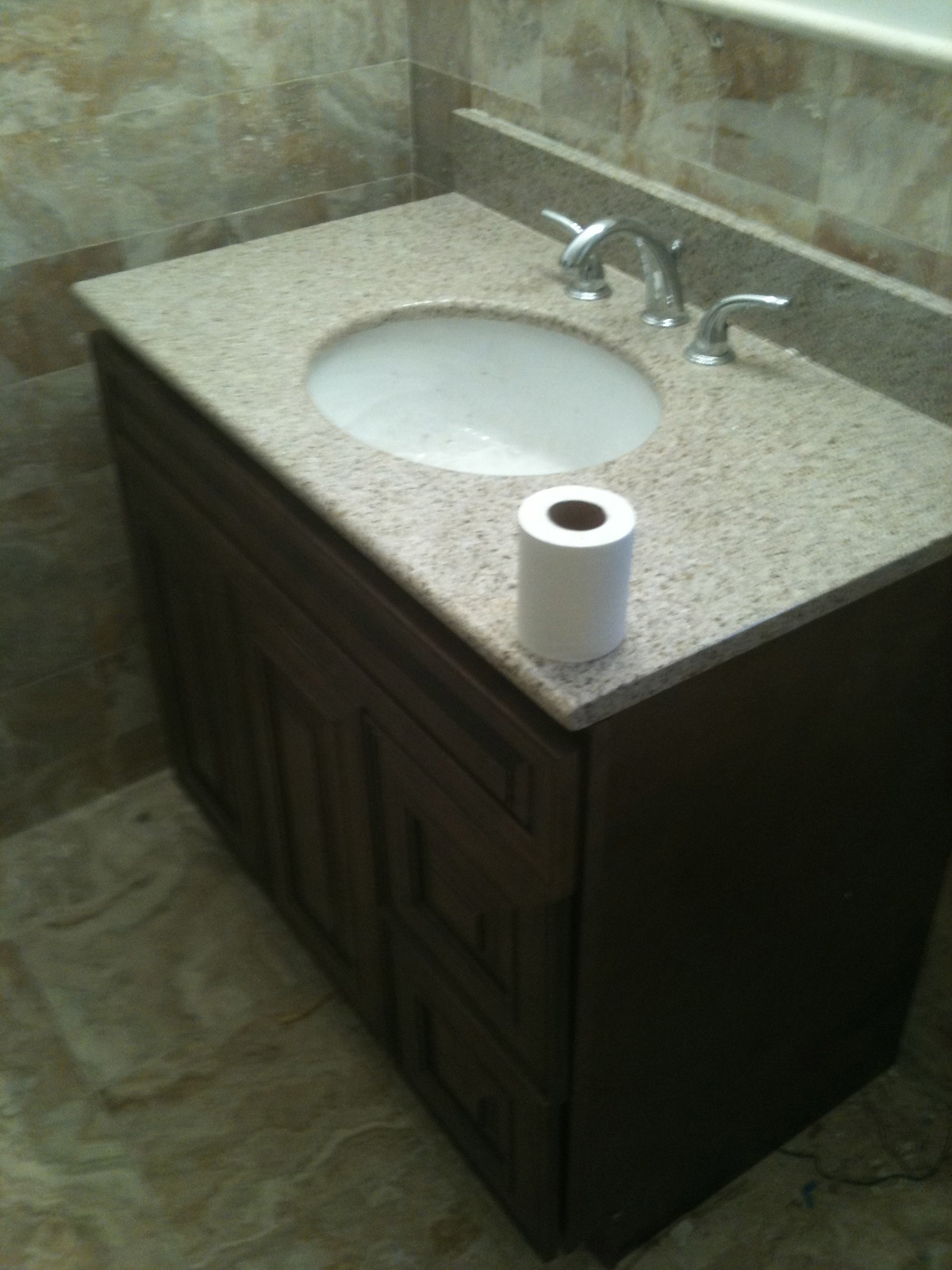The image features a bathroom vanity sink scene. In the background, there is a tiled wall, which might be either reflected in a mirror or consist entirely of tiles. Dominating the right side is the vanity unit itself, equipped with a brushed nickel faucet accompanied by two handles for hot and cold water, all converging into a single spout. The sink is a round, white marble basin, nestled into a speckled porcelain countertop. Positioned on the corner of this countertop is a partially used roll of toilet paper. The vanity unit is crafted from very dark brown wood and features doors at the front. The floor of the bathroom is also tiled, in a beige-brown shade, complementing the overall aesthetic of the space.